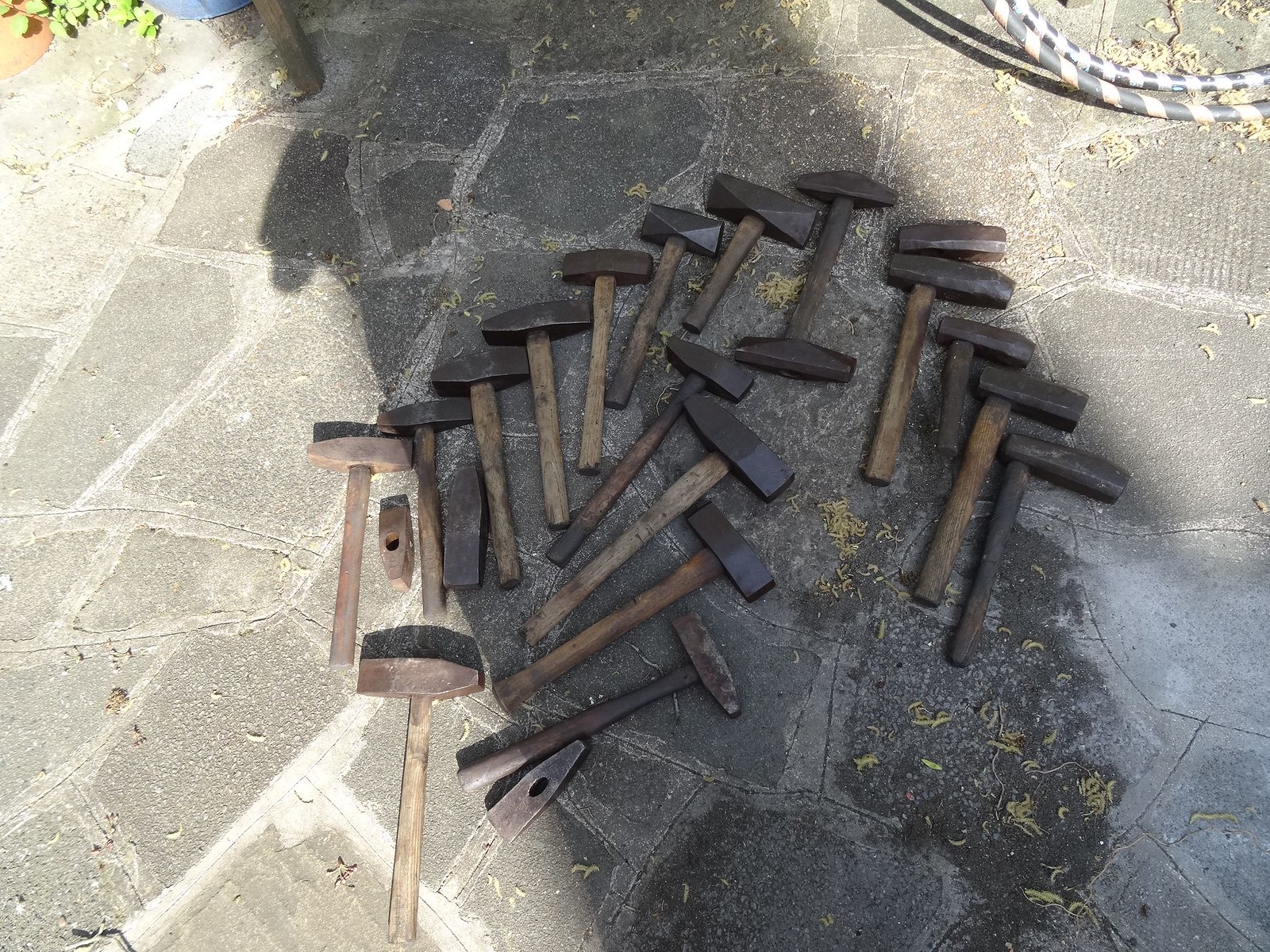The photograph depicts approximately 15 to 20 various-sized hammer mallets, arranged on a stone pavement resembling a flagstone patio under the sunlight, with some shadows cast across the tools. Each mallet features a wooden handle and a metal head, with some tapered to a point at one end and others flat. There are unique configurations as well, including double-ended tools and what appears to be a scraper. The mallets are scattered on stones of multiple shapes, which shows evidence of recent rain with drying patches and a still-wet portion. In the scene's top right corner is a black and white striped hose, while a green plant is visible in the top left. The shadow extends from the tools, partially covering them, and includes a glimpse of a person's elbow in the image's shadow. The overall appearance of the mallets is worn and aged, suggesting they are heavy-duty tools likely used in blacksmithing or metalworking.